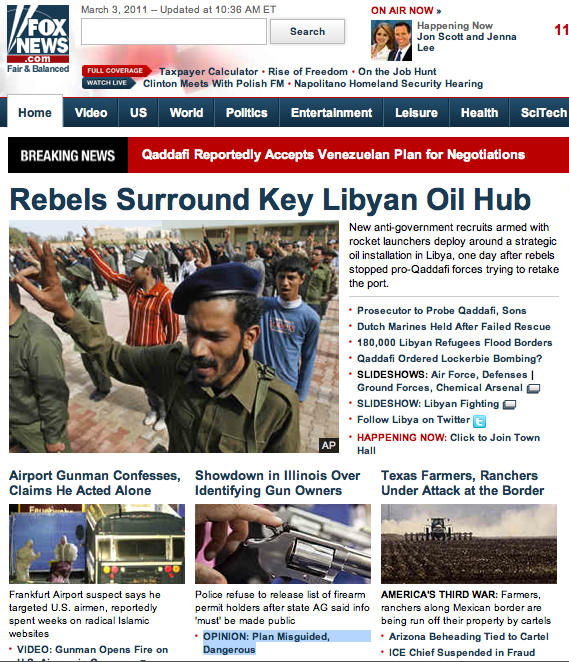In the upper left corner of the image, there is a small square displaying "foxnews.com" and a search bar beside it. Above this, the date "March 3, 2011" and the time "updated at 10:36 a.m. Eastern Time" are indicated. To the right, in red text, it reads "On Air Now," and next to this, there is a small image of a woman and a man inside a square, labeled "John Scott and Jenna Lee." Below this image, a black rectangle bears the text "Breaking News." Adjacent to it, a red rectangle states, "Qaddafi reportedly accepts Venezuelan plan for negotiations." Below this, in dark blue text, it reads "Rebels surrounded key Libyan oil hub."

The main portion of the image shows a group of people, some dressed in green military uniforms with black hats and others in regular street wear. The individuals have their mouths slightly open and their hands extended upwards towards the left, with their fingers pointed. To the side of this image, text reads, "New anti-government recruits armed with rocket launchers deploy around a strategic oil installation in Libya, one day after rebels stopped pro-Qaddafi forces trying to retake the port."